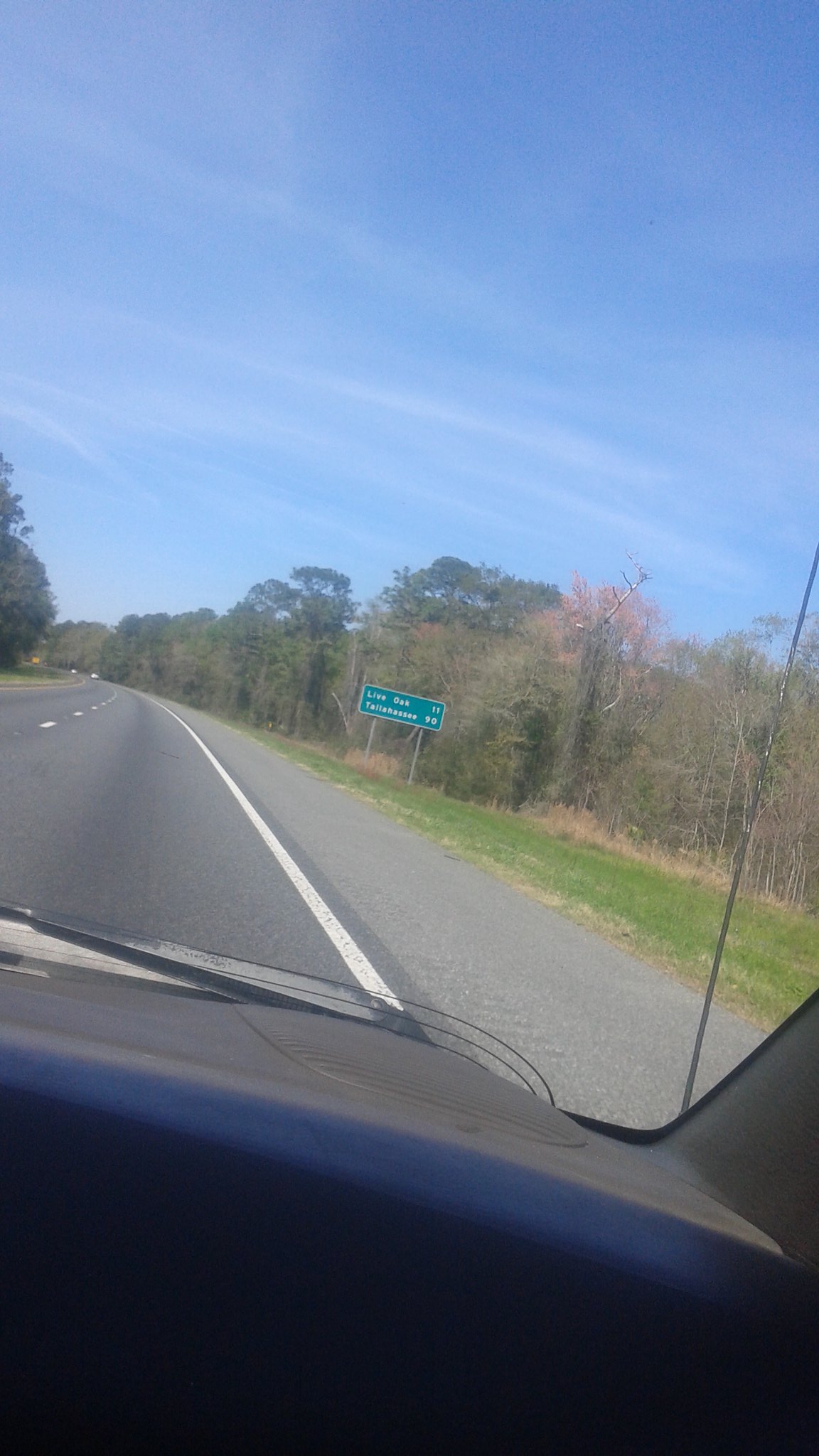A daytime photograph captured from inside a moving vehicle, providing a clear view of a well-maintained concrete road. The road features a prominent white line along one edge and a dashed white line running down the center. A green highway sign with white lettering is visible in the distance, though the text is too small to read. The roadside landscape showcases a mix of green and patchy brown grass, with a backdrop of trees. Some trees are lush with green leaves, while others are bare. The sky above is bright blue, streaked with thin, wispy white clouds. The dashboard of the vehicle is partially visible at the bottom of the frame, adding context to the perspective.